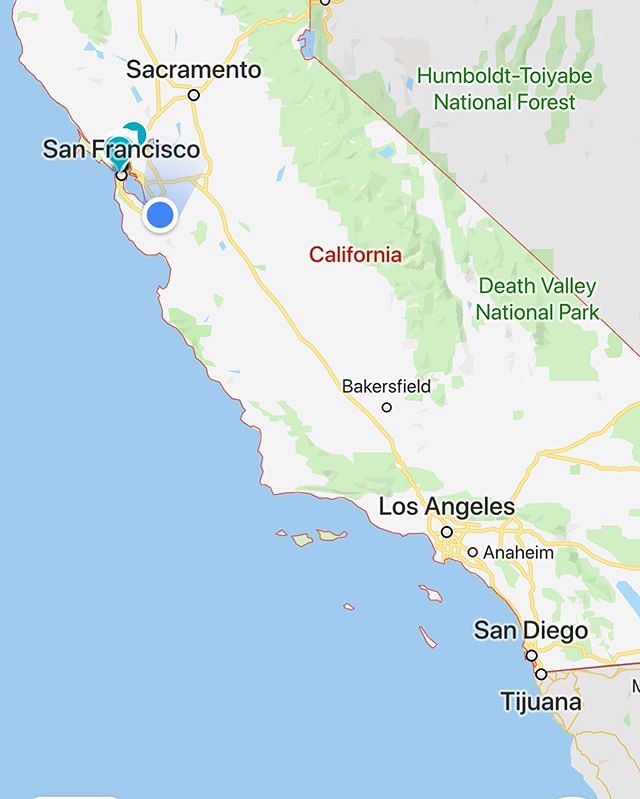The image is a detailed map of California, rendered in a rectangular shape. The state of California is depicted prominently, extending from the top to the bottom of the map, with the Pacific Ocean shaded in a light blue color occupying the bottom left, diagonally. Key cities are marked, beginning with Sacramento at the top. Moving southward, San Francisco is marked below Sacramento. In the center of the state, the word "California" is displayed in a reddish-brown text. Other cities are labeled in black font: Bakersfield, followed by Los Angeles, then Anaheim, and finally San Diego near the southern border. The map also extends slightly beyond California’s southern border to include Tijuana in Mexico. In the top right corner of the map, a gray triangle with green text labels the Humboldt-Toiyabe National Forest. Below this area, additional green shading indicates more forested regions. At the bottom right of this green section, Death Valley National Park is noted. This complex depiction of geographical and urban elements provides a comprehensive overview of California and its neighboring regions.